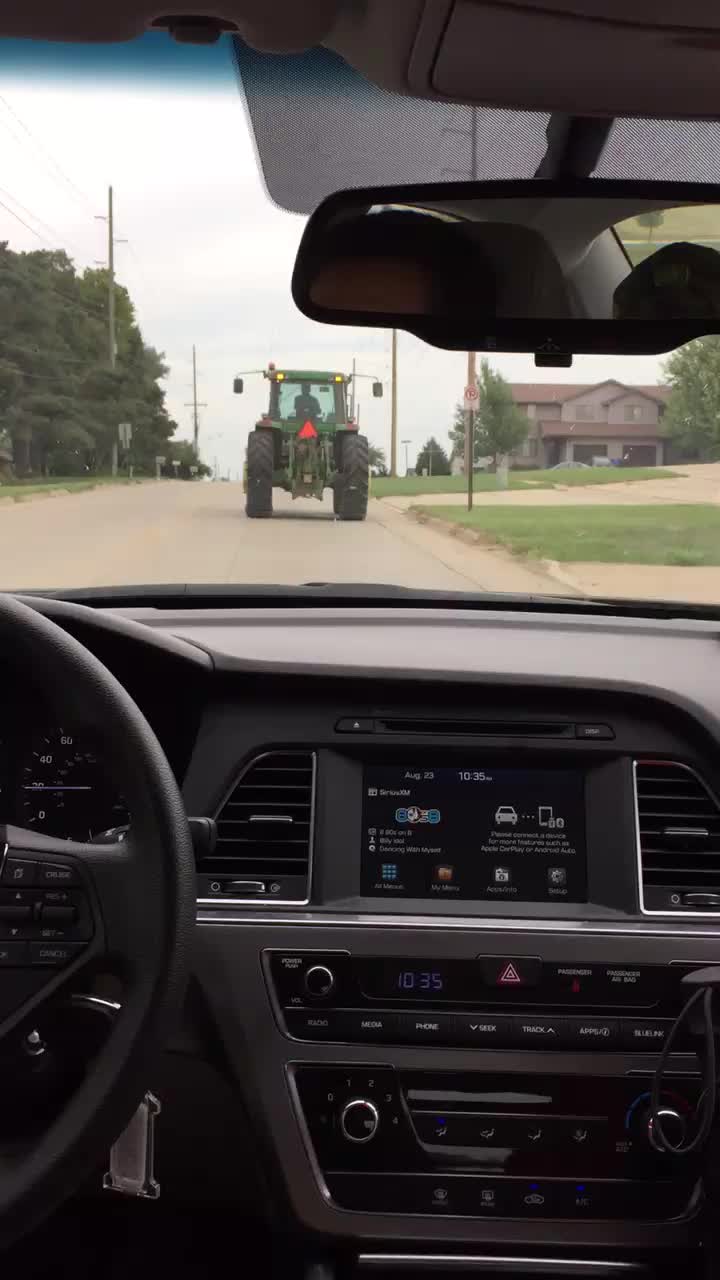The image showcases the view from inside a car, capturing the driver’s perspective. Partially visible on the left is the steering wheel, accompanied by a dashboard featuring a navigation system, radio, and CD player. A keychain dangles beneath the dashboard. Through the front windshield, a green tractor with an orange triangular sign can be seen, progressing slowly down a two-lane suburban road. Power lines flank both sides of the road, and to the right, there is a substantial, upscale two-story brick house. The sky above is predominantly white with scattered clouds, adding a serene backdrop to the suburban setting. In the rearview mirror, the reflection of a man with short hair, presumably the driver, is visible. The tractor ahead, typical for its slow speed, hints at the driver's inevitable slow-paced journey. To the left, there are several trees, and driveways leading to other homes can also be seen, further enhancing the suburban atmosphere.